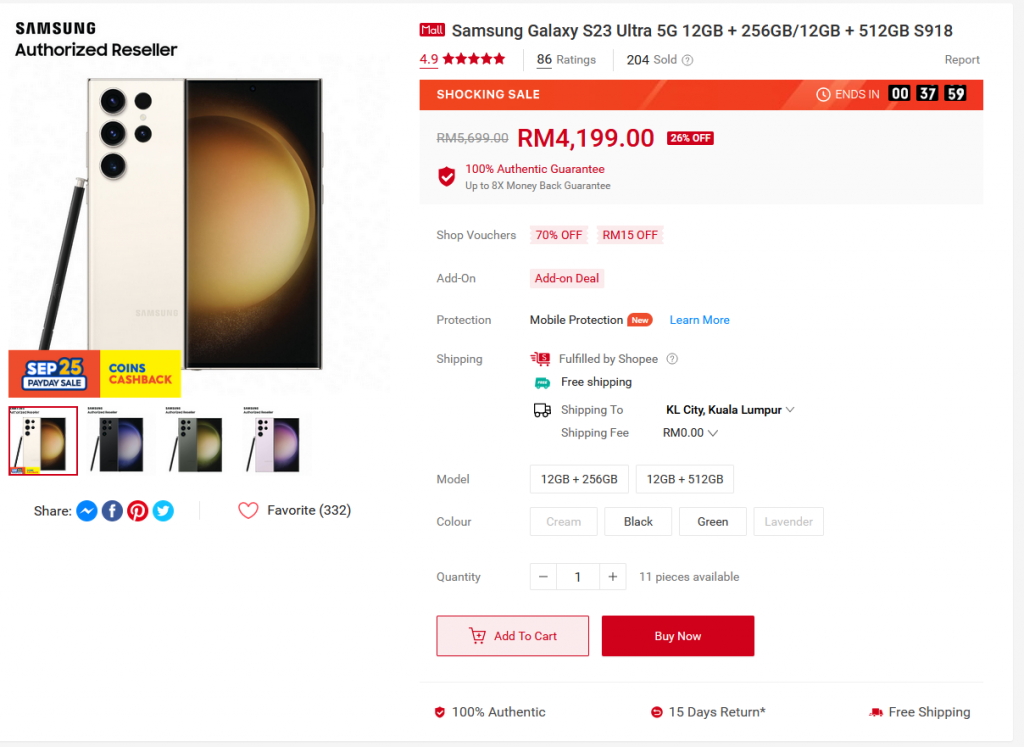This image captures a detailed view of the Samsung website, highlighting the promotion of the Samsung Galaxy S23 Ultra 5G. In the top left corner, the site designates "Samsung Authorized Reseller." Below this header, prominently displayed, is the image of a Galaxy smartphone, specifically showcasing its sleek back with three large camera lenses and two smaller ones. To the right of the camera setup, there appears to be a smaller flip display featuring an image next to the lenses. Additionally, a stylus pen is seen leaning against the phone on the left side.

Beneath the phone's image, there's a promotional banner for a "Sep 25 Friday Sale" encased in a bold red rectangle. Adjacent to this is another banner in a yellow rectangle advertising "coins cash back." The page also displays four different color variations of the phone model, each thumbnail encouraging users to explore different styles.

Furthermore, social sharing options are provided, along with social media icons. A heart symbol denotes favorites, with "332" marked beside it. The phone is identified as the "Samsung Galaxy S23 Ultra 5G," available in configurations of "12GB + 256GB" and "12GB + 512GB" (S918). The product boasts an impressive rating of 4.9 out of 5 stars based on 86 reviews and records 204 units sold.

A "Shocking Sale" banner stretches across the listing, emphasizing an extraordinary deal. The product is marked as "100% authentic," and there's additional information regarding shipping. At the bottom of the screenshot, the purchase options are visible, including a quantity selector set to "1," along with "Add to Cart" and "Buy Now" buttons in rectangular boxes.